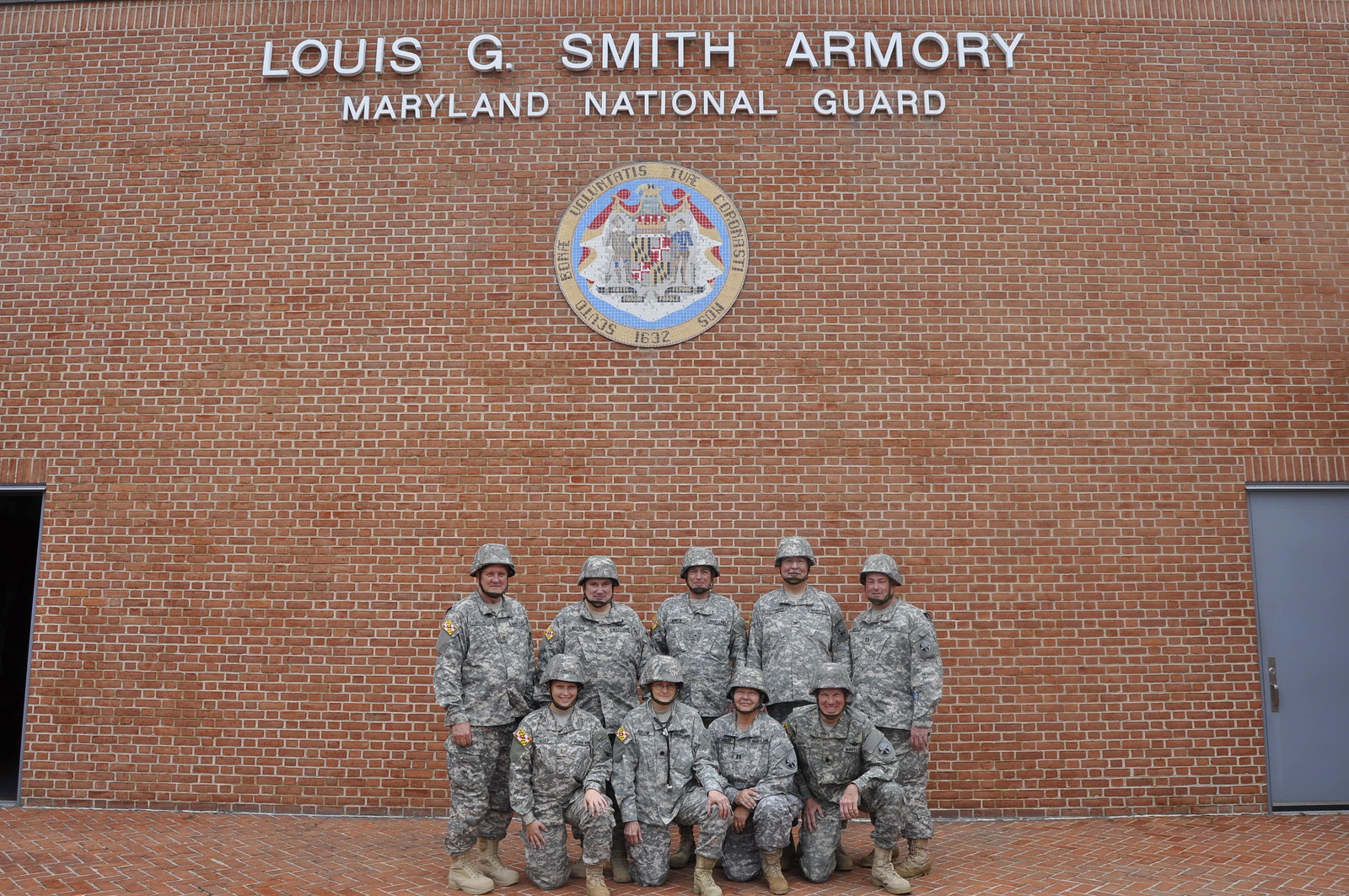In this image, a group of nine soldiers, five standing in the back and four kneeling in the front, pose for a photograph against a large red brick building. The soldiers are attired in army fatigues and helmets, with their ages varying from some who appear to be in their 20s to others who have gray hair. At the top of the building, large all-capital letters spell out "LOUIS G. SMITH ARMORY, MARYLAND NATIONAL GUARD," with the text for Maryland National Guard being slightly smaller in size. The font used is a sans-serif type that closely resembles Arial. Positioned below this text is a circular Maryland state seal, featuring the Maryland flag and surrounded by Latin inscriptions, "Scuto Bone Voluntatis Tuae Coronasti Nos 1632." The backdrop and the ground are both composed of the same red brick, offering a cohesive and historical setting for the photograph.